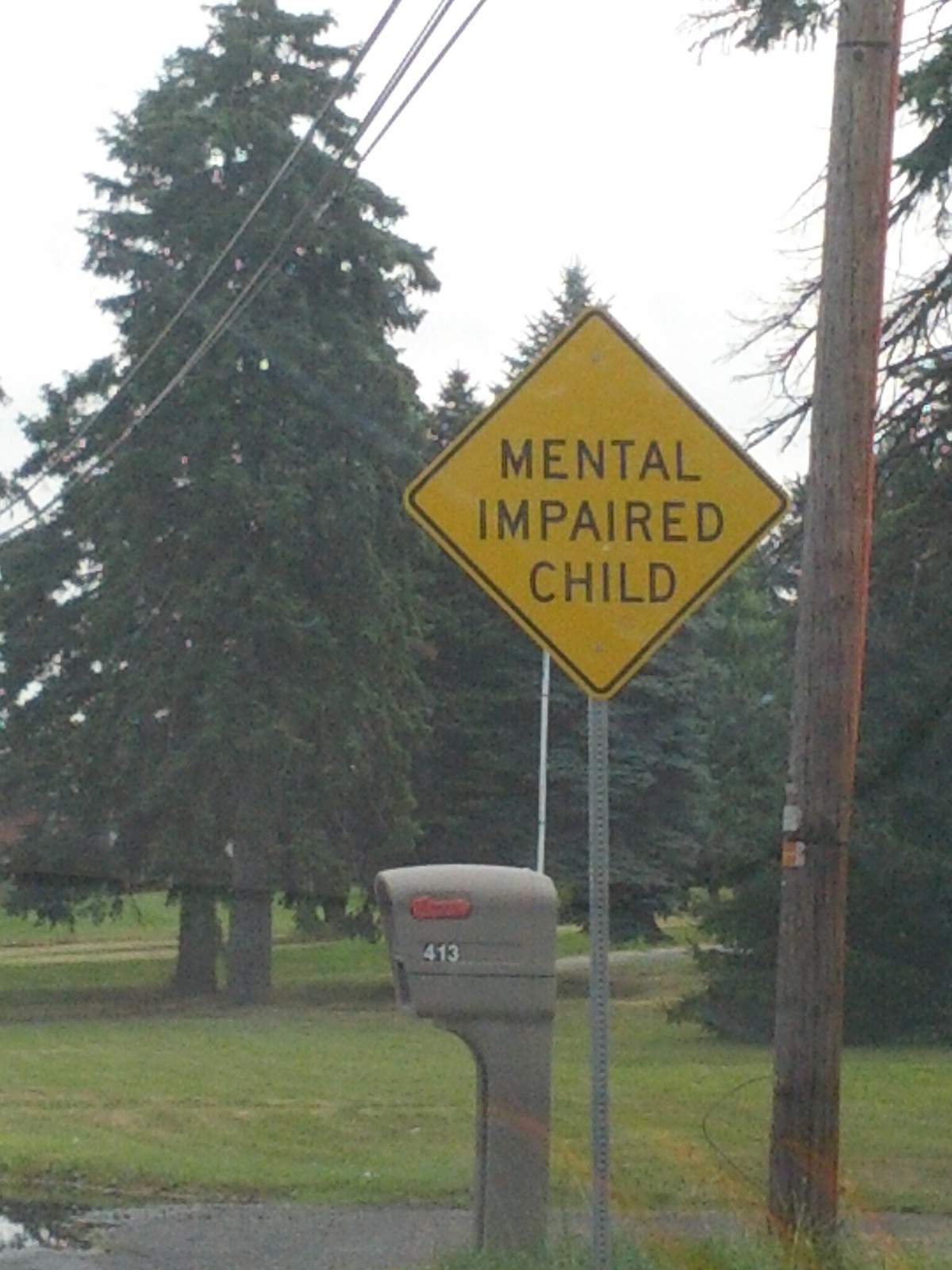This outdoor image depicts the entrance to a residential neighborhood under a gloomy, gray sky. Dominating the foreground is a light gray mailbox bearing the street number 413 in white, with its red flag lowered. Just behind the mailbox stands a warning sign for a "Mental Impaired Child," diamond-shaped and yellow with black lettering and a border, mounted on a silver post. To the right of these is a telephone pole with several metal tags and power lines extending from the upper center to the middle left of the image. The background reveals a paved street partially visible at the bottom, bordered by well-manicured green grass and an array of very tall evergreen trees, including a prominent cedar fir. The scene captures a quiet neighborhood seemingly poised for attention to the specific caution indicated by the sign.